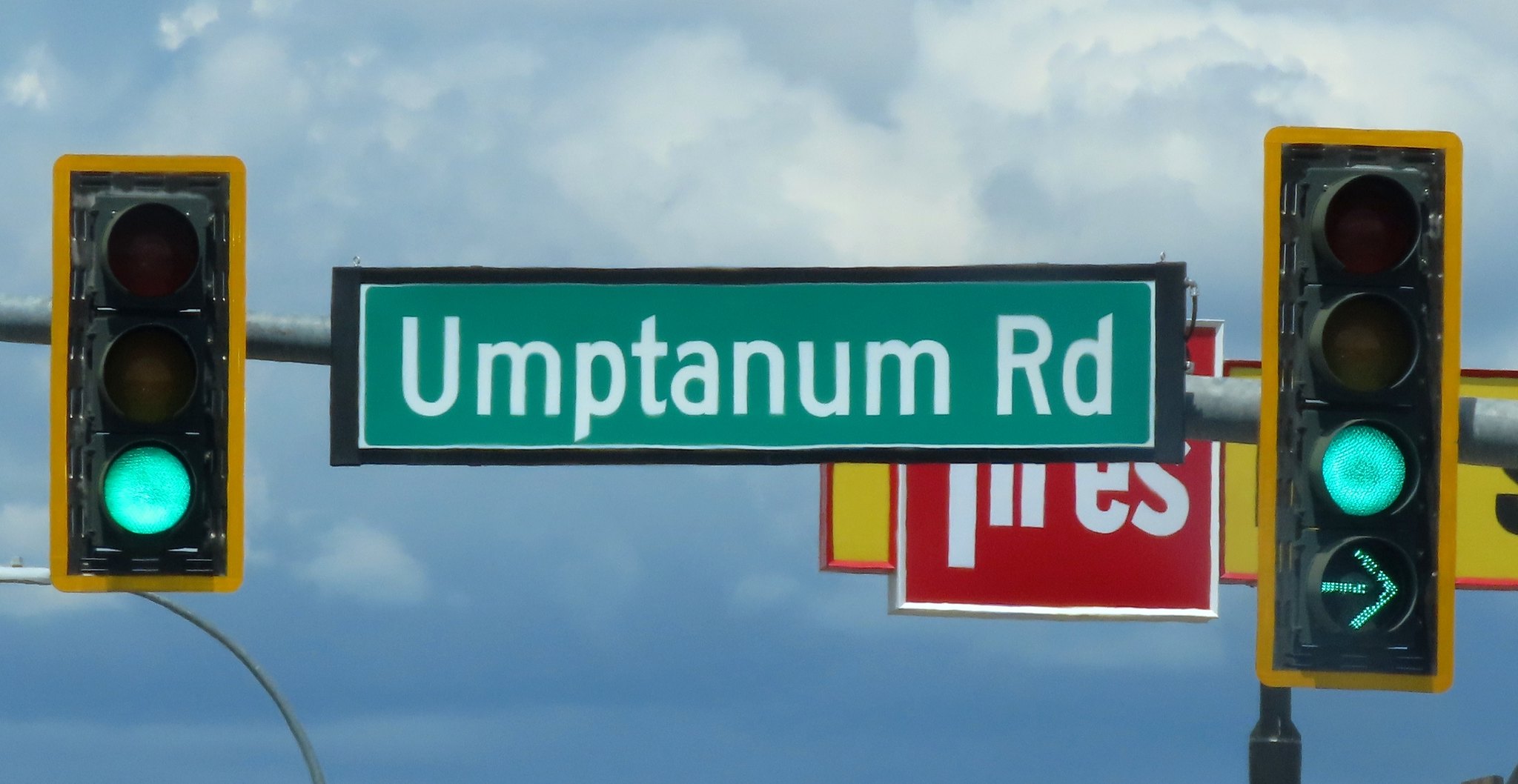The photograph captures a green street sign reading "Canum Rd" in white letters, flanked by two traffic lights. The left traffic light consists of four signals, displaying a green light and a green arrow beneath it. The right traffic light, although also showing a green light, has only three signals without an arrow. In the background, a partially visible red sign with the letters "ES" appears cut off, making its full text indecipherable. The backdrop of this urban scene features a clear blue sky adorned with fluffy white clouds, indicating pleasant weather. The street is devoid of any pedestrians, contributing to the serene atmosphere of the photograph.